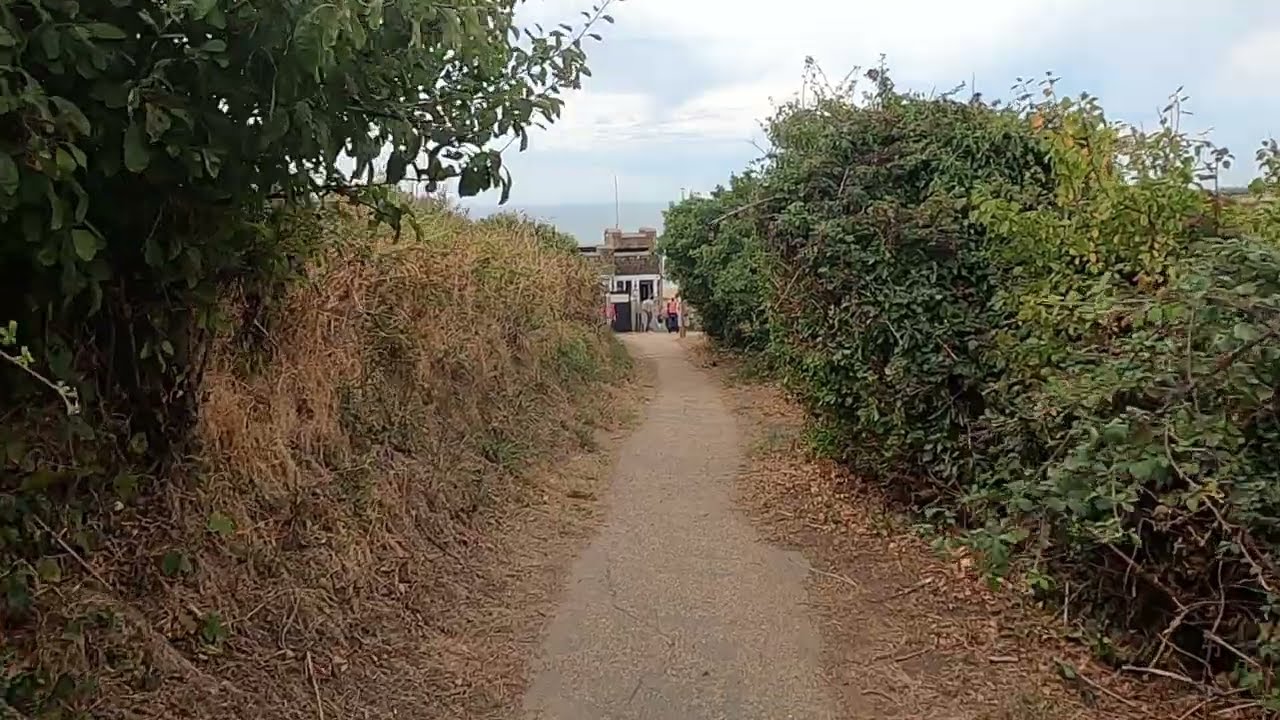The image captures a picturesque countryside scene featuring a narrow cement path, just wide enough for a person to walk, leading towards a rectangular white building with a gray roof. The path, central to the composition, is flanked by walls of various bushes on both sides, interspersed with dead leaves. In the top portion of the image, a light blue sky with scattered white clouds creates a tranquil backdrop. There is a subtle suggestion of a mountainous area, hazy in the distance, lending a sense of depth to the scene. 

At the end of the road, partially hidden by the plant walls, we see the white building with an antenna or flagpole extending from its top. In front of this building stand several people, including one wearing a black shirt with tan pants and another in black pants with a pink shirt. The scene is bathed in natural daylight, indicating that the photo was taken outdoors in the middle of the day. The setting evokes a serene, rural atmosphere, possibly suggesting a pathway leading to a beach or another area beyond the building.